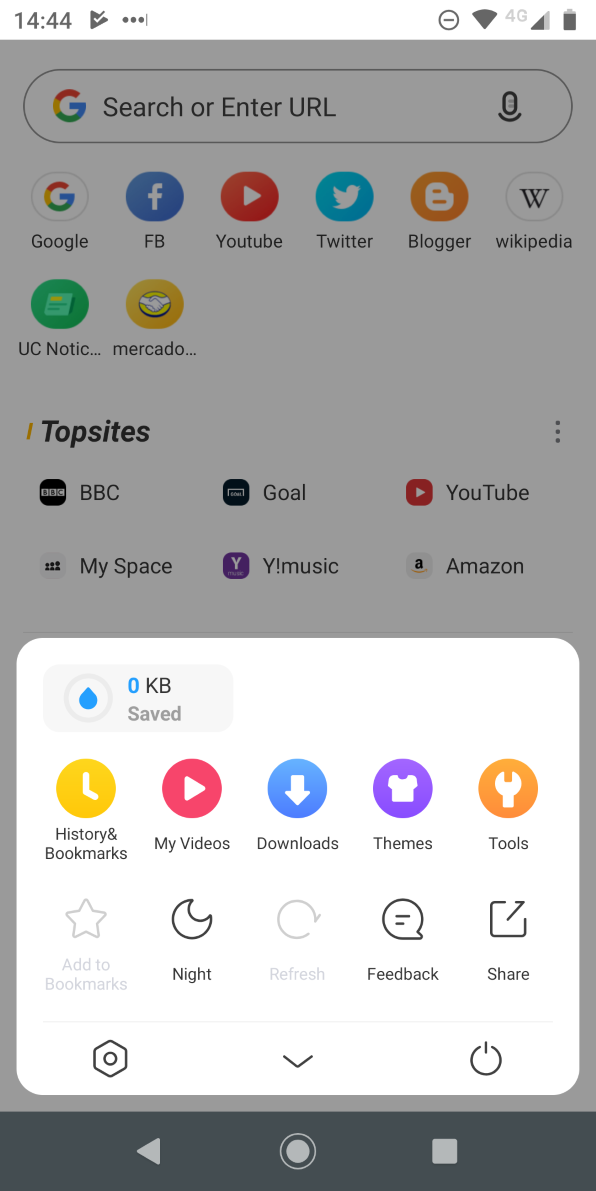The image depicts a mobile phone screen with a highly detailed interface. The background of the screen is grayed out, bringing the foreground into sharp focus. 

At the top of the screen, there's a white status bar displaying the time "14:44," indicating 2:44 PM. This bar includes three circular icons, a triangle with a checkmark inside, and a minus sign encased in a circle. It also shows the phone is connected to a 4G network, the battery is nearly full, and the signal strength is strong.

The grayed-out background features the Google search bar with its distinctive multicolored "G" logo, offering the option to "search or enter URL." Next to the search bar, there's a microphone icon for voice-activated search.

Beneath the search bar are several recognizable app icons: 
- Google (multicolored "G"),
- Facebook (blue circle with a white "F"),
- YouTube (red circle with a white play button),
- Twitter (blue circle with a white bird),
- Blogger (orange "B"),
- Wikipedia ("W"),
- UC Notifications, 
- Mercado.

Below these icons is a section titled "Top Sites," listing links to BBC, Goal, YouTube, MySpace, Why Music, and Amazon.

Dominating the foreground is a white box showing a water drop symbol encased in a circle, marked with "0 KB saved." Below this marking, there are a series of icons and options:
1. **History and Bookmarks:** Yellow circle with a white clock face showing 4 o'clock.
2. **My Videos:** Red circle with a white play button (similar to the YouTube icon).
3. **Downloads:** Blue circle with a downward arrow.
4. **Themes:** Purple circle with a white t-shirt.
5. **Tools:** Orange circle with a wrench symbol.
6. **Add to Bookmarks:** Grayed out icon of a star.
7. **Night Mode:** Grayed out moon icon.
8. **Refresh:** Grayed out circle with an incomplete arrow.
9. **Feedback:** Speech bubble.
10. **Share:** Paper icon with an arrow pointing to the upper right.
11. **Additional Menu:** A hexagon with a circle in the middle and a downward arrow.
12. **Power Button:** An icon for on/off functionality.

This detailed interface reflects a comprehensive and user-friendly mobile experience, neatly categorizing functions and frequently-used sites and features.